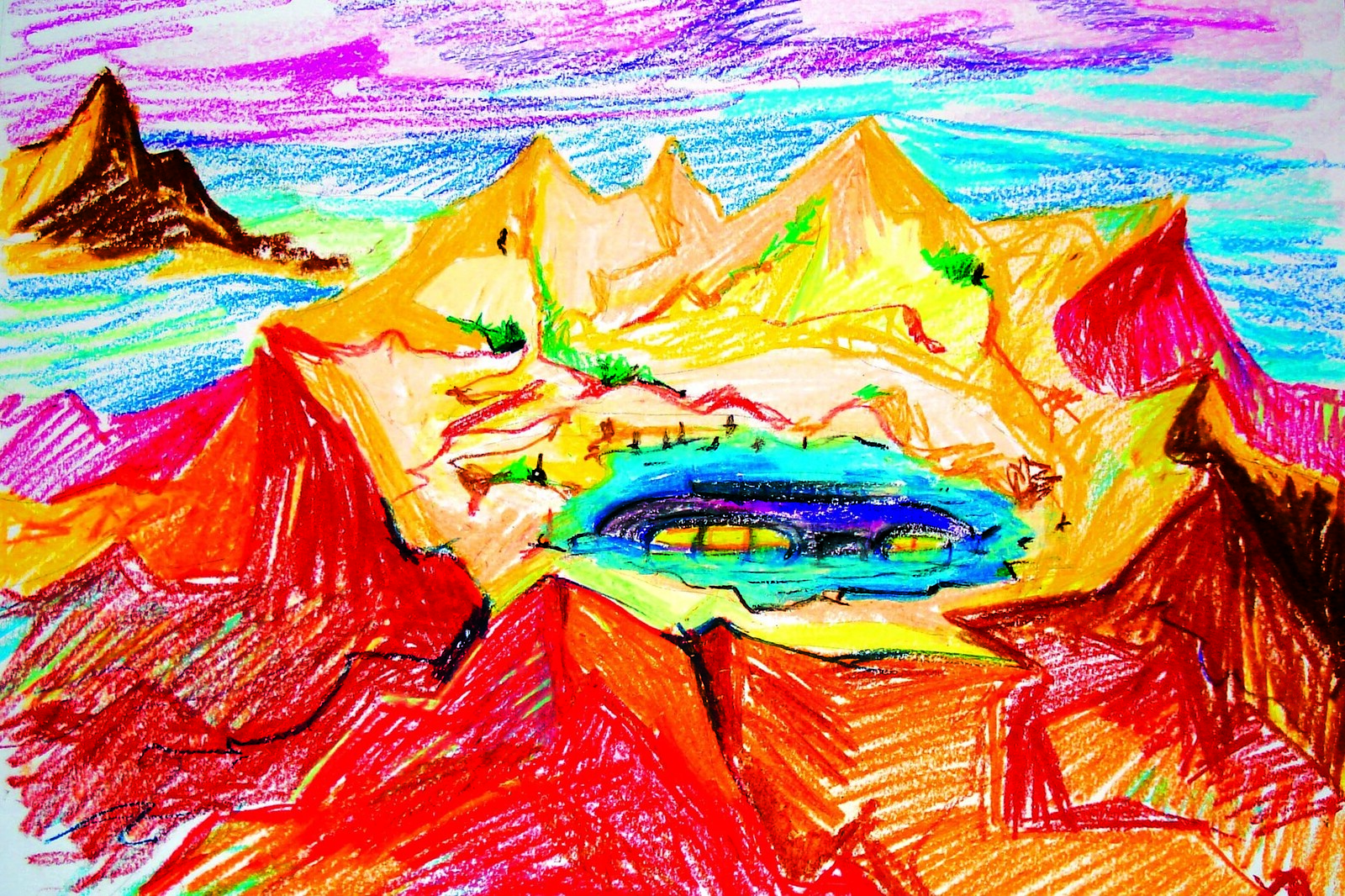This vibrant artwork features a central, oval-shaped body of water resembling a lake, rendered in a vivid blend of green, blue, and yellow hues. This lake is nestled within a striking, volcano-like crater characterized by its jagged, spiky terrain in rich shades of red, orange, and yellow. Scattered throughout the scene are patches of lush green grass and various plant life, adding a touch of natural serenity. Above, the sky is awash in dramatic purples and blues, creating a dreamlike atmosphere. In the background, a distant mountain with a smooth, rounded peak rises majestically into the sky, completing the breathtaking landscape.